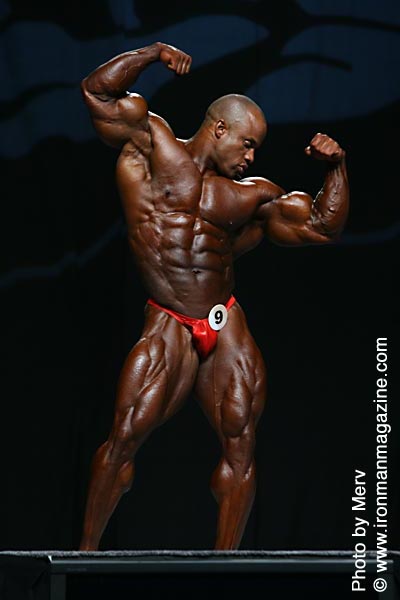The image depicts an African-American male bodybuilder performing on stage during a competition. He is wearing a red posing suit, commonly referred to as a g-string or Speedo, which features a yellow circle with a black number nine, likely his contestant number. The bodybuilder is bald or has a very short haircut and is striking a flexing pose with his right arm raised higher than his left, while his head is turned towards his left bicep. His physique is highly muscular and well-defined, showing no visible fat. The background is predominantly black with some gray hues. In the bottom right corner of the photograph, white text reads "photo by Merv" with the website "www.ironmanmagazine.com." The entire scene is well-lit and serves to highlight the bodybuilder's form and definition.